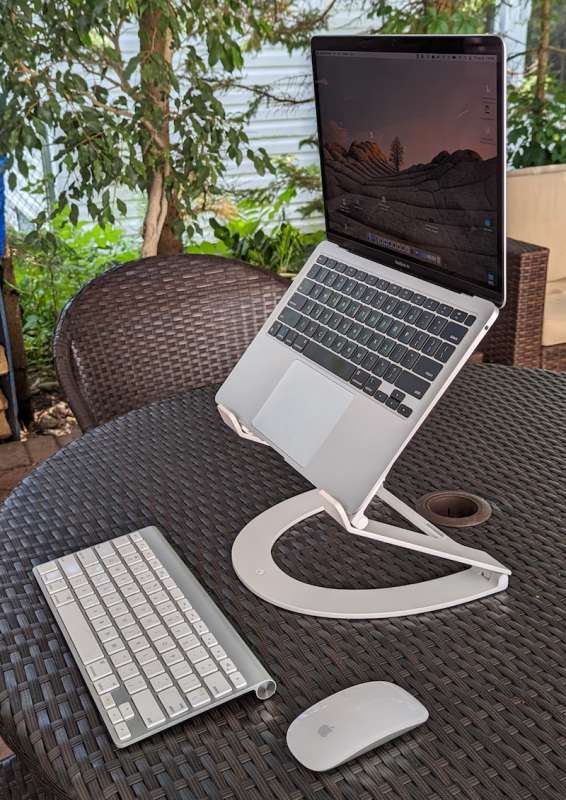This photograph, taken during the day, features a silver Apple laptop with a black screen and keys, positioned on a white, C-shaped, arch-like stand. The laptop, which has a screensaver of a landscape with a hill and a tree, is elevated at an angle on a black wicker table. In front of the laptop, there is a gray Apple keyboard with white keys and darker gray in between, as well as a white Apple mouse. The table, which has a hole in the center presumably for an umbrella, is situated in a garden porch setting. Surrounding the table are a black wicker chair on the left and a matching brown wicker sofa with tan cushions in the background. Lush greenery, including trees and plants, along with a glimpse of a white house, frames the serene outdoor space.